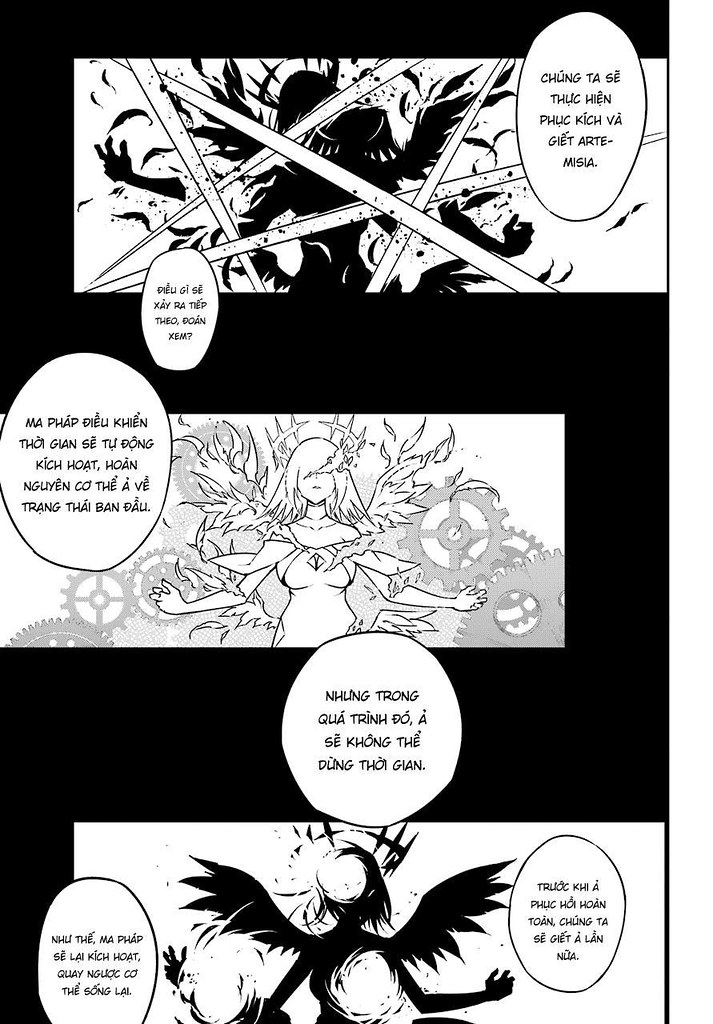This black-and-white illustration is a page from a foreign comic magazine, divided into three horizontal panels against a dark background. The top panel depicts an intense battle scene with several swords slicing through a black monster, creating an explosive burst of lines resembling a star, and scattered with hints of blood and body parts. The middle panel features a woman striking a powerful pose with outstretched arms, surrounded by swirling flames and metallic gears framing her, suggesting an enigmatic, supernatural aura. In the bottom panel, the woman reappears as a dark silhouette, as if transformed, commanding orbs of energy or fireballs around her, amidst a shadowy atmosphere. This stylized sequence conveys dramatic and mystical elements, embodying the graphic, dynamic storytelling typical of comic art.